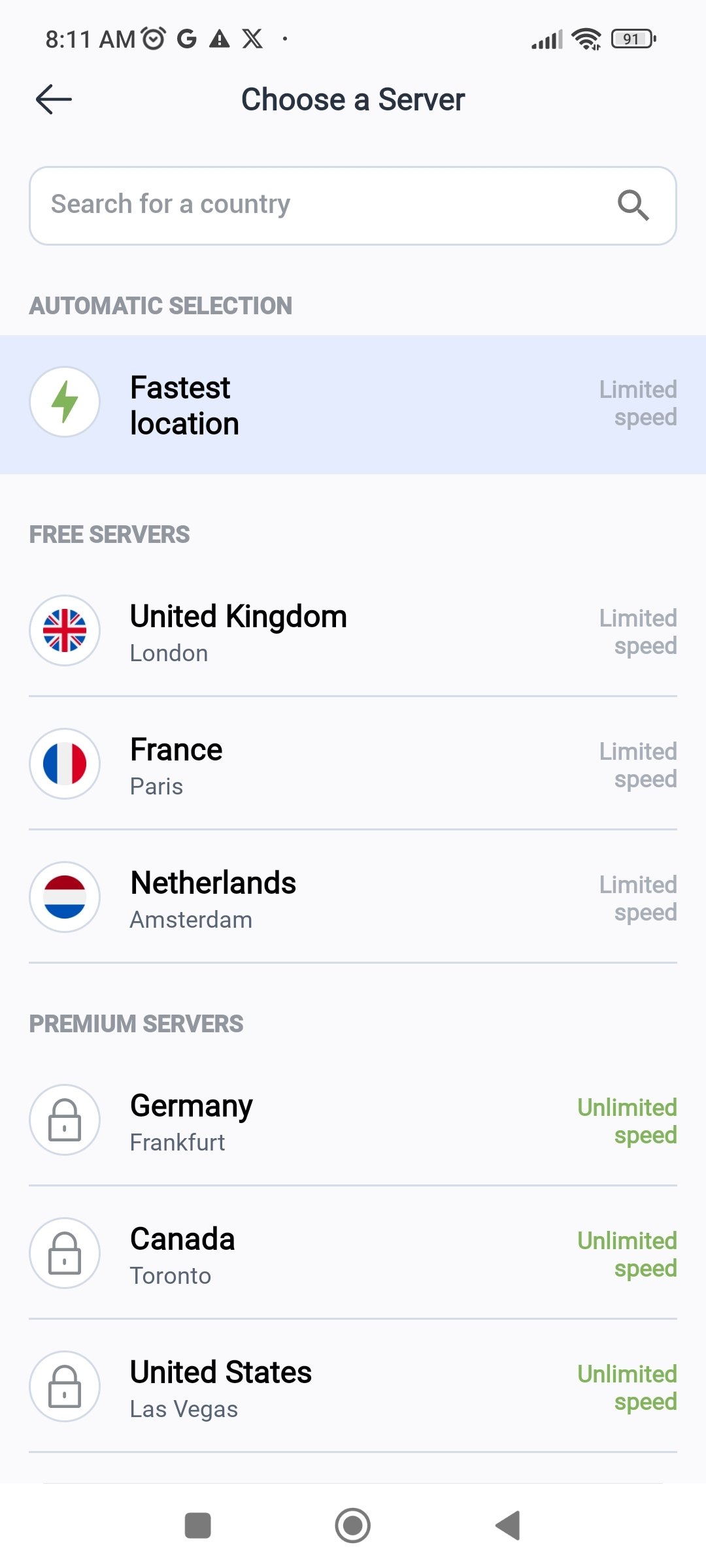A screenshot captured on a cell phone displays a "Choose a Server" page within an unidentified application featuring a white background. At the top, bold text reading "Choose a Server" is prominent. Beneath this heading, there is a search bar labeled "Search for a country." Below the search functionality, the "Automatic Selection" option is highlighted with a blue bar, indicating it has limited speed and is the currently selected server.

Further down, the "Free Servers" section lists available options, each accompanied by location details and speed limitations:
- United Kingdom, London (Limited speed)
- France, Paris (Limited speed)
- Netherlands, Amsterdam (Limited speed)

Following the free servers, the "Premium Servers" section showcases options, each marked with a lock symbol within a white circle to denote restricted access and offering unlimited speed:
- Germany, Frankfurt
- Canada, Toronto
- United States, Las Vegas

The "Fastest Location" server is currently selected, as indicated by the blue bar, but it also notes limited speed capabilities.